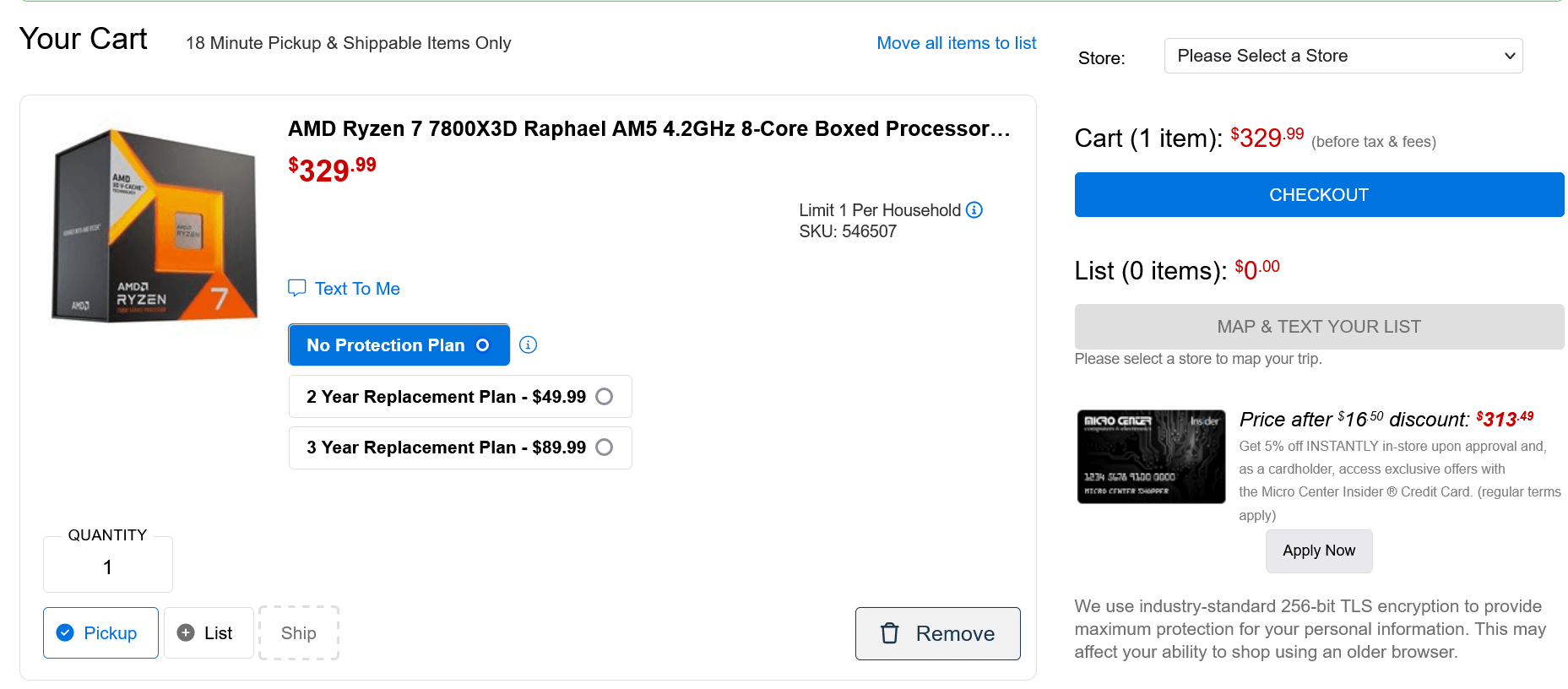This is a screenshot from a desktop PC depicting an online shopping cart. The website's name is not visible, but the page title reads "Your Cart" at the top left-hand corner. The user has added one item to the cart: an AMD Ryzen 7 7800X3D Rafale AM5 boxed processor. This 8-core processor operates at 4.2 GHz and is priced at $329.99. The cart offers the option to include a protection plan, with choices of a two-year plan for $49.99 or a three-year plan for $89.99. Alternatively, the user can opt out of purchasing a protection plan. There is a note indicating a limit of one processor per household, and the user has selected the option to pick up the item in-store.